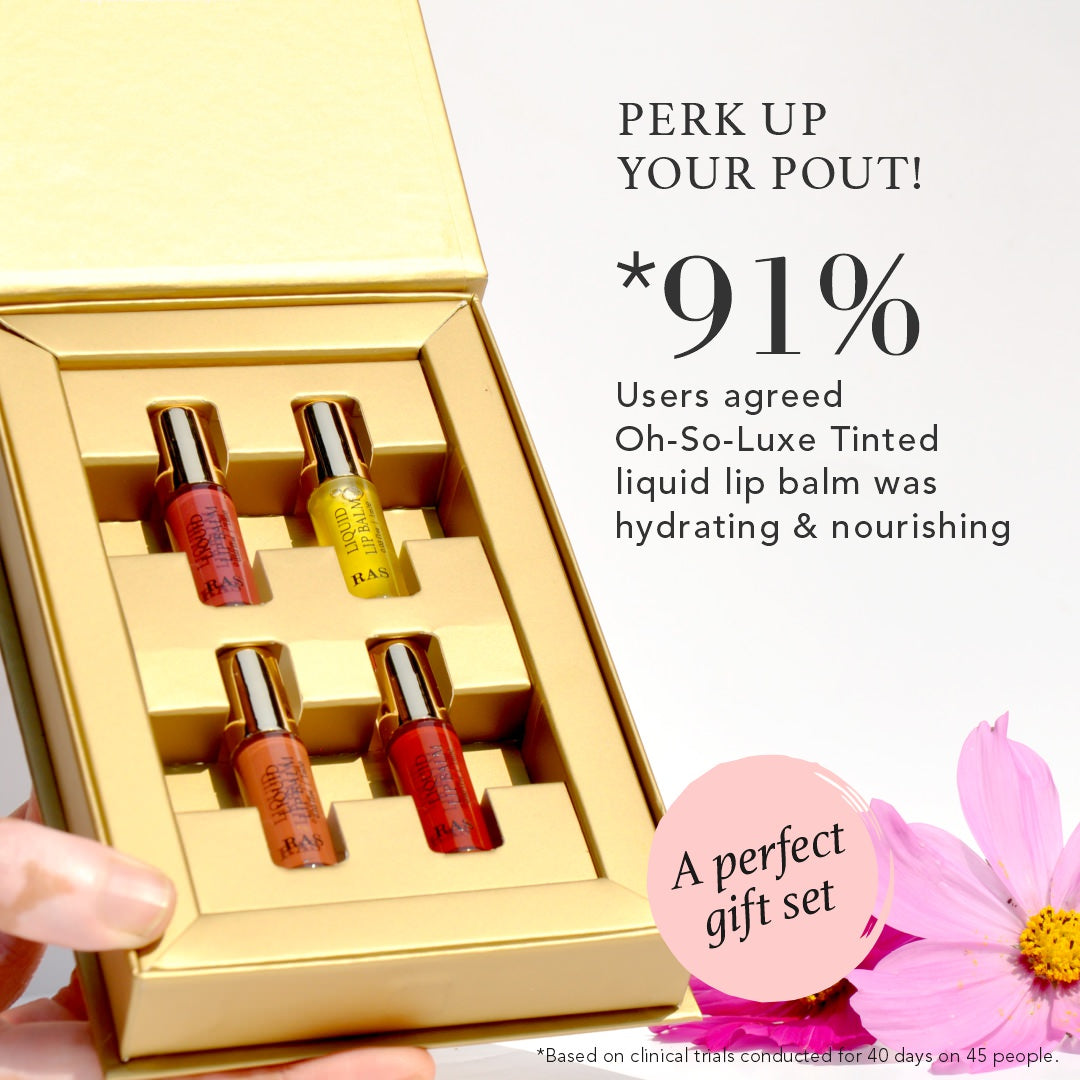This image is an advertisement for Oh So Luxe Tinted Liquid Lip Balm, set against an off-white background. Central to the image is a gold, rectangular gift box with the lid open, being held at an angle by a visible hand. The box contains four small glass bottles of lip balm, each topped with a gold cap. Arranged in the box, starting from the upper left is a red lip balm, followed by a yellow one to its right. Below these are an orange lip balm on the left and a darker red balm on the right. 

On the right side of the image, bold black text reads, "Perk up your pout," followed by "91%" in larger text. Beneath that, it states, "Users agreed Oh So Luxe Tinted Liquid Lip Balm was hydrating and nourishing," with an asterisk referring to a note at the bottom. There, smaller text adds, "*Based on clinical trials conducted for 40 days on 45 people."

Additionally, in the lower right corner, there is a pink circle with black text stating, "A perfect gift set," accompanied by two flowers - a bright pink flower with a yellow center, and a darker pink flower positioned slightly behind it, adding a touch of elegance and softness to the overall look of the advertisement.